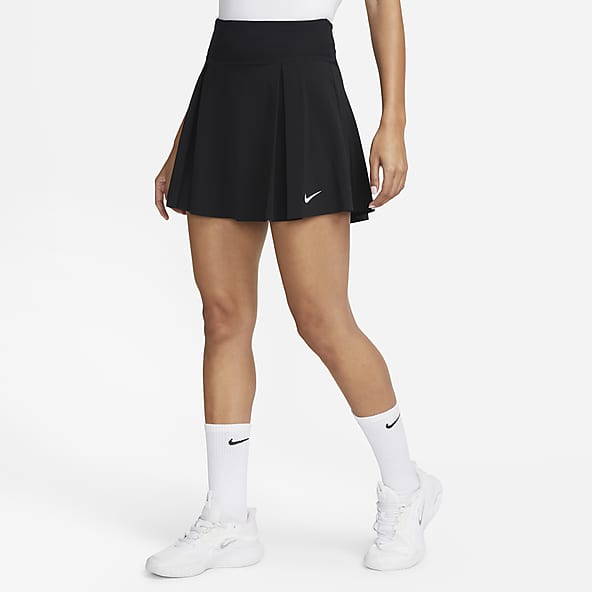The image depicts a model from the waist down against a plain white background. The model is wearing a white shirt tucked into a black, slightly pleated, Nike skirt that flares out, with the Nike swoosh logo visible just above the right thigh. Their arms rest by their sides, fingertips reaching the bottom of the skirt. The model adopts a walking pose, with the left leg slightly behind the right. She sports white mid-calf Nike socks, featuring black swoosh logos on the sides, and white Nike sneakers with matching white shoelaces. The combination of attire suggests a youthful and sporty aesthetic.